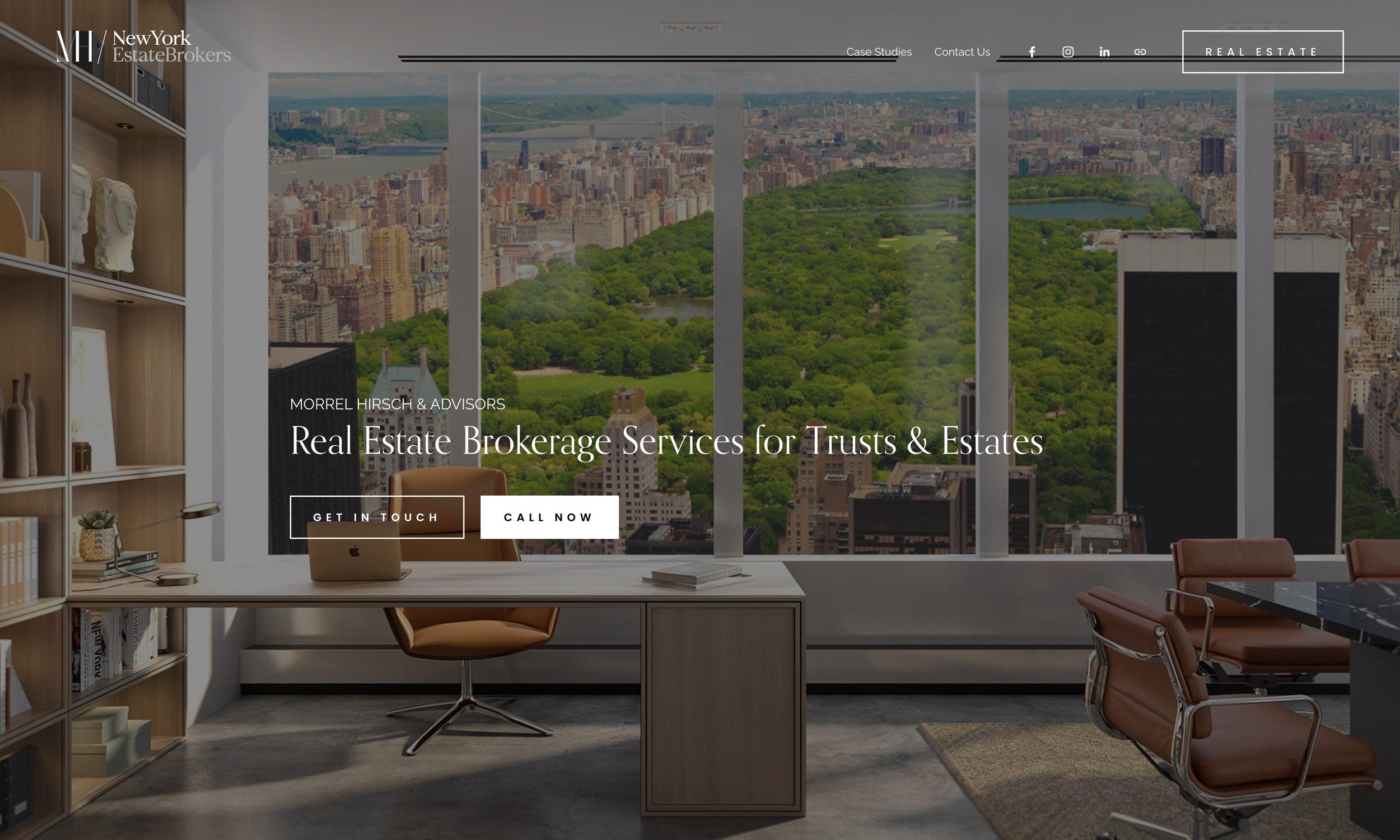This web page, representing New York Estate Brokers, prominently features a photograph of a sleek, modern office setting. In the upper left-hand corner, the company's logo appears with the capital letters 'M' and 'H,' followed by a slash, and then 'New York Estate Brokers' in white text. 

Across the top of the page to the right, navigation options include 'Case Studies,' 'Contact Us,' and several social media icons—Facebook, Instagram, LinkedIn, and an unidentified icon. Below these options is a distinct white rectangle featuring the words 'Real Estate.'

The photograph dominating the page showcases an ultra-modern office with sophisticated desks and chairs. Large, nearly floor-to-ceiling windows encompass the space, granting a panoramic view of New York City's urban landscape. These windows frame several panels separated by white beams, giving an expansive look at both the city skyline and a large green space, presumably Central Park. Beyond this, a body of water is visible.

Centrally placed in this photograph, bold white text reads, 'Real Estate Brokerage Services for Trusts and Estates.' Above this, in smaller white text, the names 'Morrel Hirsch and Advisors' are displayed, signaling the firm's specialized focus within the real estate sector.

This composition effectively conveys an image of sophistication and expertise in New York's competitive real estate market.